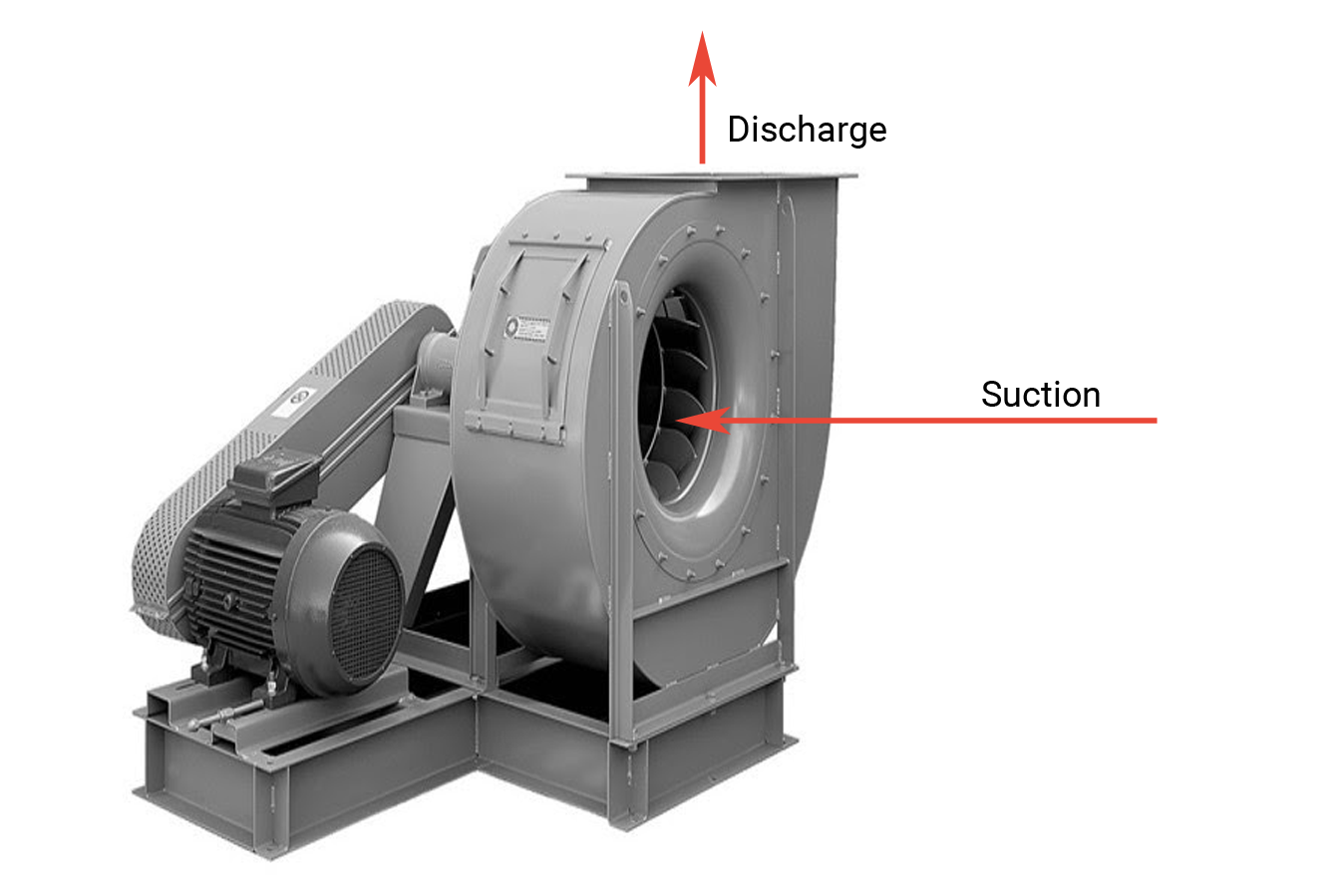The image features a large, industrial, gray air purifying system or mechanical device, prominently marked with labels and arrows indicating its functional areas. This robust machine includes a substantial cylindrical component, possibly a fan, clearly marked by a red arrow labeled "suction" in black lettering at the front. The "suction" area features an opening that seems designed to intake materials. On the opposite side, a red arrow points upwards to an opening labeled “discharge,” indicating where processed material exits, akin to a chimney. The device also has a motor connected by what appears to be a series of gears or a conveyor belt, mounted on large metallic blocks. It sits against a stark white background and white wall, emphasizing its substantial size and industrial nature.